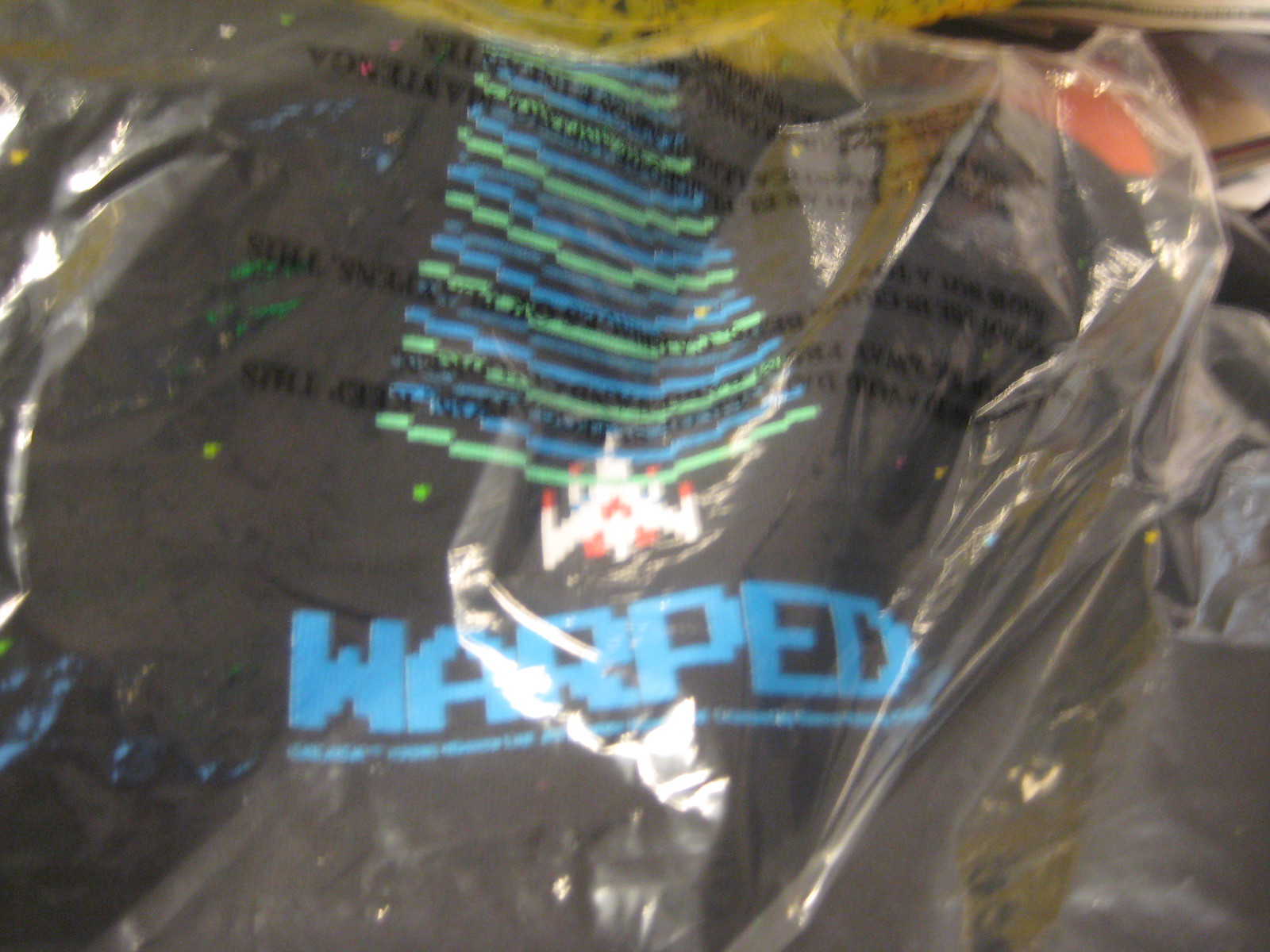The image depicts a blurry photograph of a dark-colored piece of clothing, possibly a black t-shirt, wrapped in clear cellophane packaging. Across the packaging, there is a prominent logo that says "warped" in large, blue voxel or pixelated font reminiscent of Minecraft. Above the word "warped" is a small white spaceship icon. The shirt inside the packaging appears to have a pixelated design on the back near the neck and a logo with yellow and blue striped patterns on the front. The background of the photo is dark, with some folded items visible, adding to the overall indistinct quality of the image.